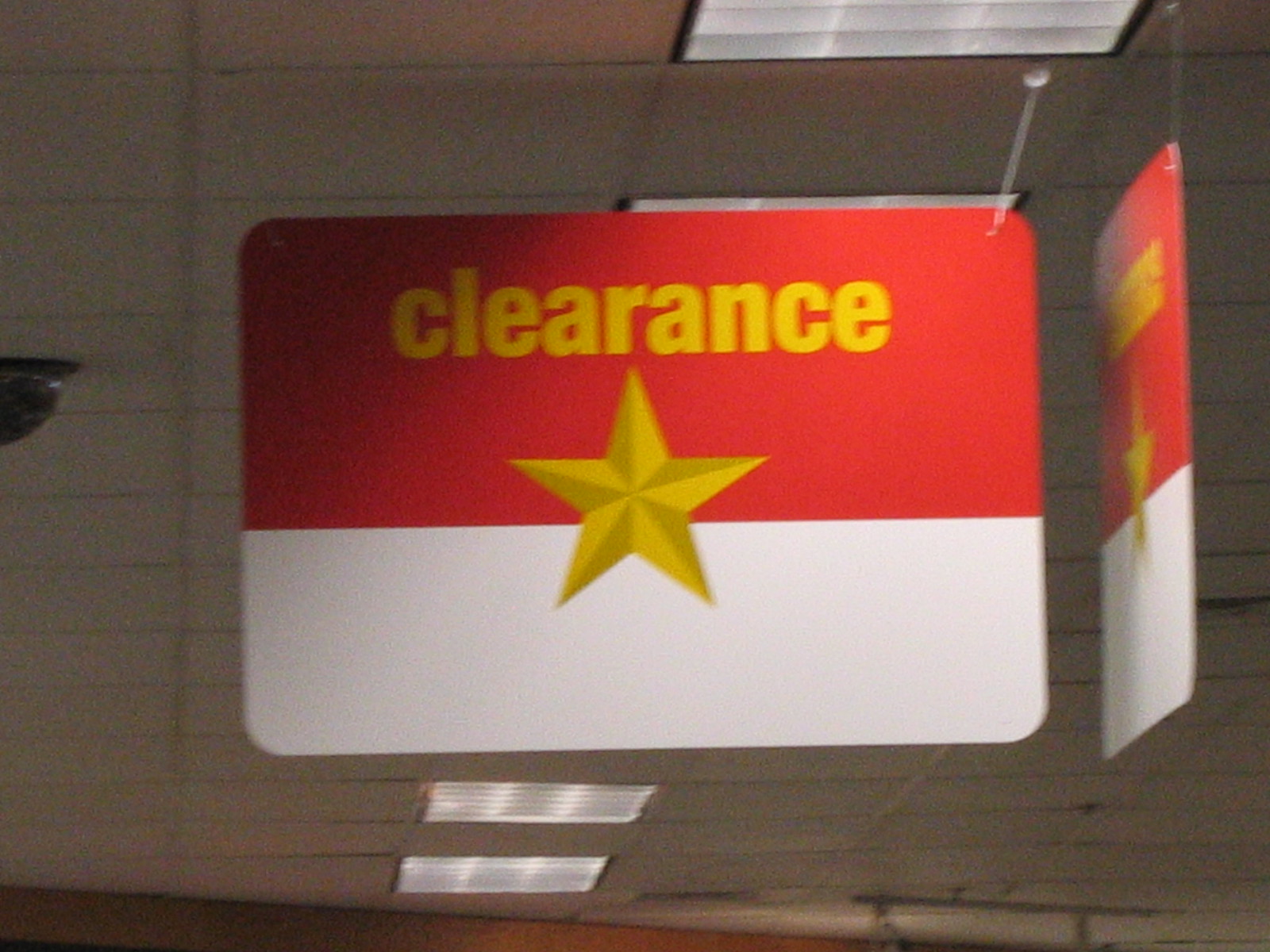The image depicts a vast space with a very tall ceiling, which stretches so high it is barely discernible. Along the entire height of the front wall are an array of pictures, arranged in a 3x3 grid. To the left side of the image, a black spherical security camera is positioned, observing the area. At the front of the space, a prominent red rectangle captures attention, adorned with yellow text that reads "square." Centrally within this rectangle, there is a star design, surrounded by lines or points radiating outward. The points on the right half of the star are yellow, while those on the left half are brown. The lower portion of the wall features a white area. Additionally, to the right, there is another sign similar to the red rectangle but oriented 90 degrees away from the viewer. The lower part of the image becomes increasingly blurred, showing more ceiling tiles and lighting fixtures receding into the distance.